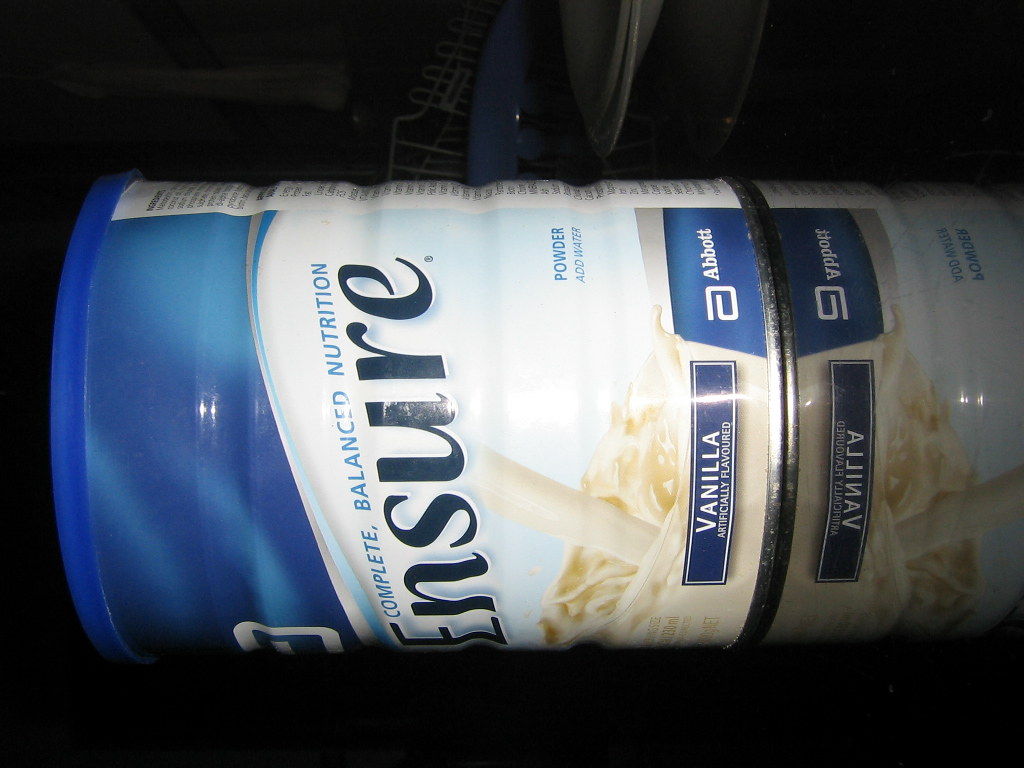In this angled image, a variety of elements create a complex yet intriguing scene. The background features a drainage ditch with several plates placed beside it, suggesting a makeshift or perhaps impromptu setting. A rag is notably draped over what appears to be the edge of a drawer, adding a sense of casual disarray. Dominating the right side of the picture is a gleaming black tabletop, its polished surface capturing reflections with striking clarity. Among the reflections, a jar of Ensure formula prominently stands out. The jar is identifiable by its blue lid and label that reads "Ensure Complete Balanced Nutrition, Vanilla, Artificially Flavored, Powder, Add Sugar, Abbott," with a distinctive blue strip above a white one. The light, emanating from an off-picture source, illuminates the scene, casting a soft glow on the jar and enhancing the overall composition of the photograph.